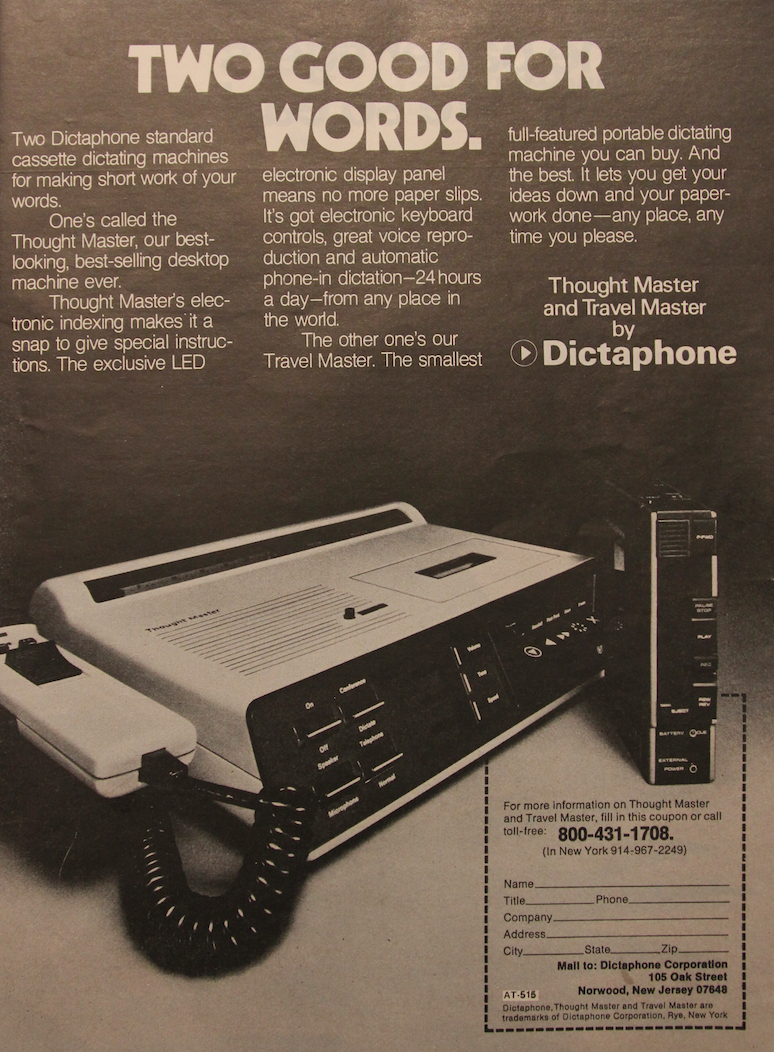This is a sepia-toned, black-and-white photographic advertisement for Dictaphone's dictating machines, featured in a likely indoor setting, resembling an old-fashioned newspaper page. The headline, "Too Good for Words," introduces two distinct models: the Dot Master and the Travel Master. 

The Dot Master is described as the best-looking and best-selling desktop machine, equipped with electronic indexing for special instructions, an exclusive LED electronic display panel eliminating the need for paper slips, electronic keyboard controls, superb voice reproduction, and automated phone and dictation capabilities 24 hours a day, from anywhere in the world. The photograph displays the Dot Master as a gray rectangular box with an inclined edge, a speaker, and a tape slot, connected to a phone.

Beside it, the Travel Master, lauded as the smallest full-featured portable dictating machine available, is designed for flexibility, allowing users to record their ideas and complete paperwork anytime, anywhere. It is shown as a small black rectangular device.

The bottom right corner features an order coupon for more information or to make a purchase, directing potential customers to fill out their details or call toll-free 800-431-1708, or 914-967-2249 if in New York. The coupon includes fields for personal and company information and addresses Dictaphone Corporation at 105 Oak Street, Norwood, NJ 07648. The advertisement reinforces the product names and trademarks of Dictaphone Corporation, Rye, New York, and invites visits to www.dictaphone.com.